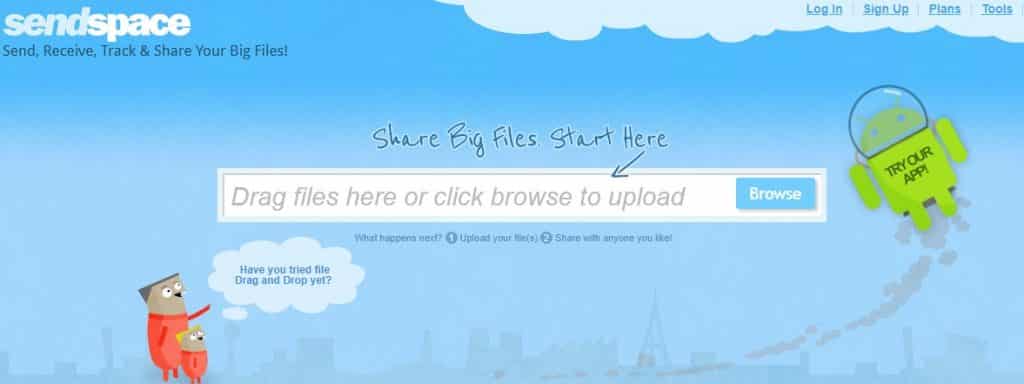The image displays a detailed section of the Sendspace website, oriented in a landscape, almost panoramic, view. The top portion of the image is dominated by a bright blue background, which transitions to a slightly lighter blue at the bottom. 

In the top left corner, the website's name, "sendspace," is prominently displayed in bold, lowercase letters with "send" in italicized white font, while "space" remains in a standard white font. Beneath the website name, in a smaller, dark blue font, the tagline reads: "send, receive, track & share your big files!" 

From the middle to the top right corner, a cloud-like shape stretches across the screen. This cloud has a white or pale blue hue and contains four blue, underlined clickable links: "Login," "Signup," "Plans," and "Tools."

Centrally located on the page, both horizontally and vertically, is a prominently placed white search bar. Above the search bar, a handwritten style font declares, "Share big file start here," with an arrow pointing down towards the bar. Within the search bar, in gray italic text, it instructs users to "drag files here or click browse to upload." On the right side of the search bar, a blue button with white font reads "Browse."

To the right of the search bar stands a small green Android figure, wearing a bubble-like spaceman helmet with the words "TRY OUR APP" emblazoned on his chest in all caps.

In the bottom left corner, a whimsical cartoon featuring two characters, possibly depicting a father and son, is shown. Their figures are blob-shaped with flat heads, dressed in red unipiece suits, and possessing big googly eyes. A speech bubble emerges from this cartoon, written in a playful, cloud-like style, which says, "Have you tried file drag and drop yet?"